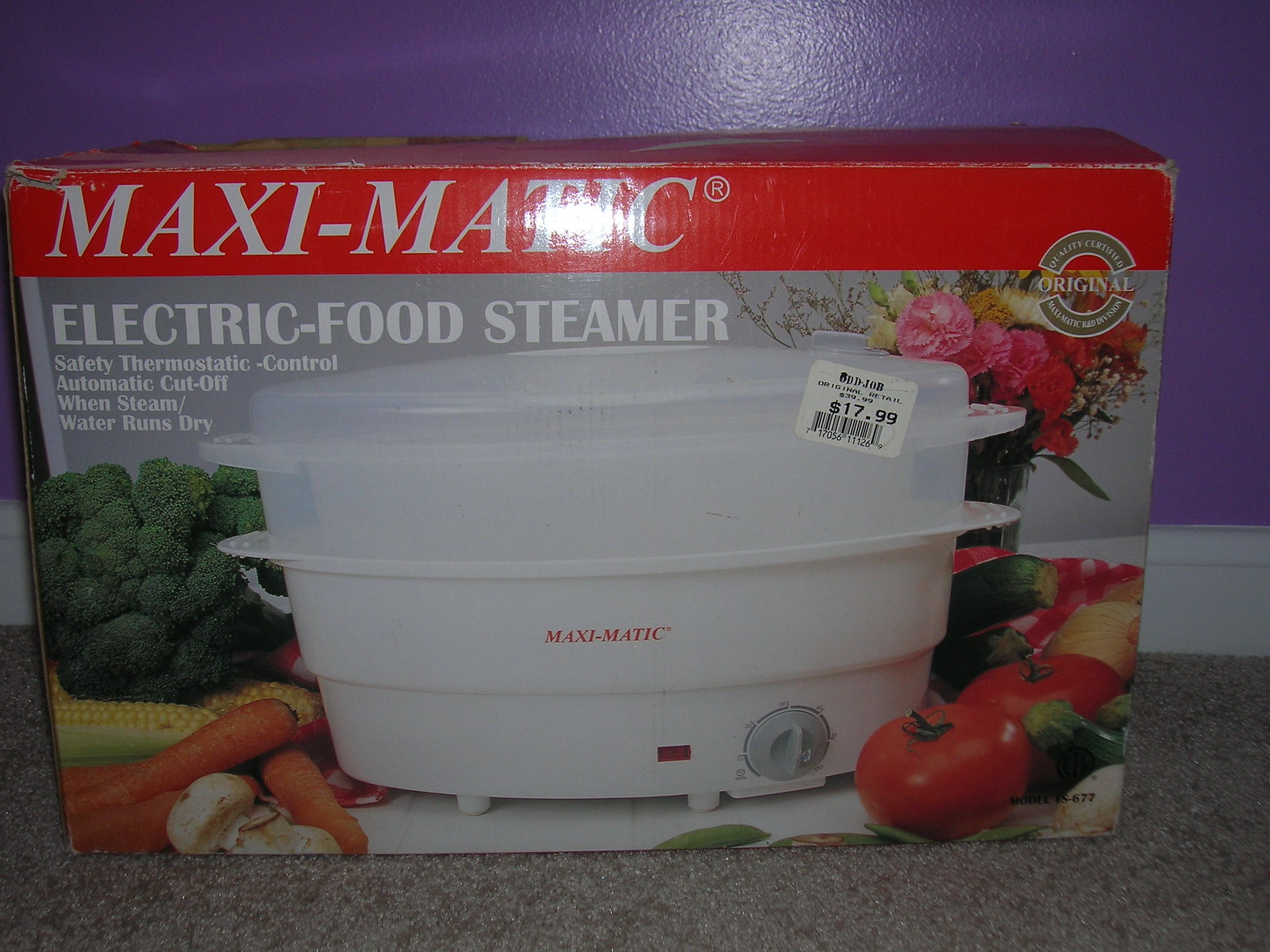This detailed photograph features a Maxi-Matic electric food steamer in its box, evocatively placed on a counter with a gray and brown speckled surface. The box is designed with a prominent red stripe at the top, showcasing the brand name "Maxi-Matic" in bold white letters. Beneath this stripe, in white lettering, it announces "Electric Food Steamer." The central image on the box depicts the white plastic steamer, which closely resembles a slow cooker but serves the purpose of steaming food. 

Highlighted in small red lettering on the steamer is "Maxi-Matic," complemented by a functional gray dial for temperature control on the lower right, along with a red indicator light to signal when the unit is operational. Surrounding the steamer on the box are vibrant illustrations of fresh vegetables, including red tomatoes, green zucchini, orange carrots, yellow corn, green broccoli, and colorful carnations in pink and yellow, hinting at the variety of foods that can be prepared using the steamer.

The box rests in a setting with a floor of light brown hue and a purple wall behind it, bordered by a white baseboard. There's also a white price tag on the box, marked $17.99. The packaging's detailed and inviting presentation captures the essence of the product, ready to attract shoppers from a store shelf.